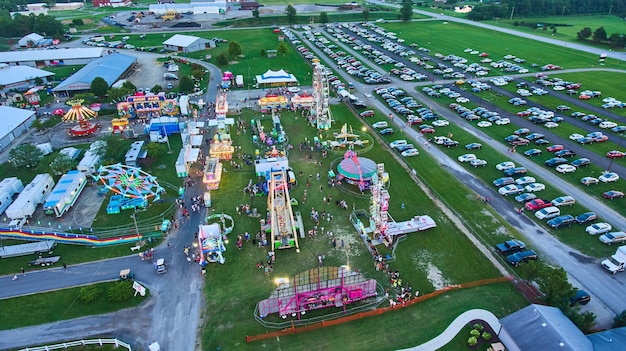The image is an aerial photograph, possibly taken from a drone, airplane, or a high carnival ride, capturing an expansive view of a county fair set in a grassy field at dusk. The vivid colors of the carnival rides—blues, reds, yellows, and neons—are coming alive as the lighting begins to take effect. The fairground is dotted with various rides, including a blue Tilt-A-Whirl on the left, a red and yellow merry-go-round, and a grand Ferris wheel. Surrounding the carnival is a sprawling grassy parking lot with paved lanes, filled with cars. To the left, there are some buildings, including barns and other farm-like structures. Portable trailers, likely used by the Kearneys, are scattered around, along with tents—presumably food stalls and game booths—adding to the colorful, bustling atmosphere. The scene captures the juxtaposition of vibrant carnival excitement against the serene, wide-open country setting.